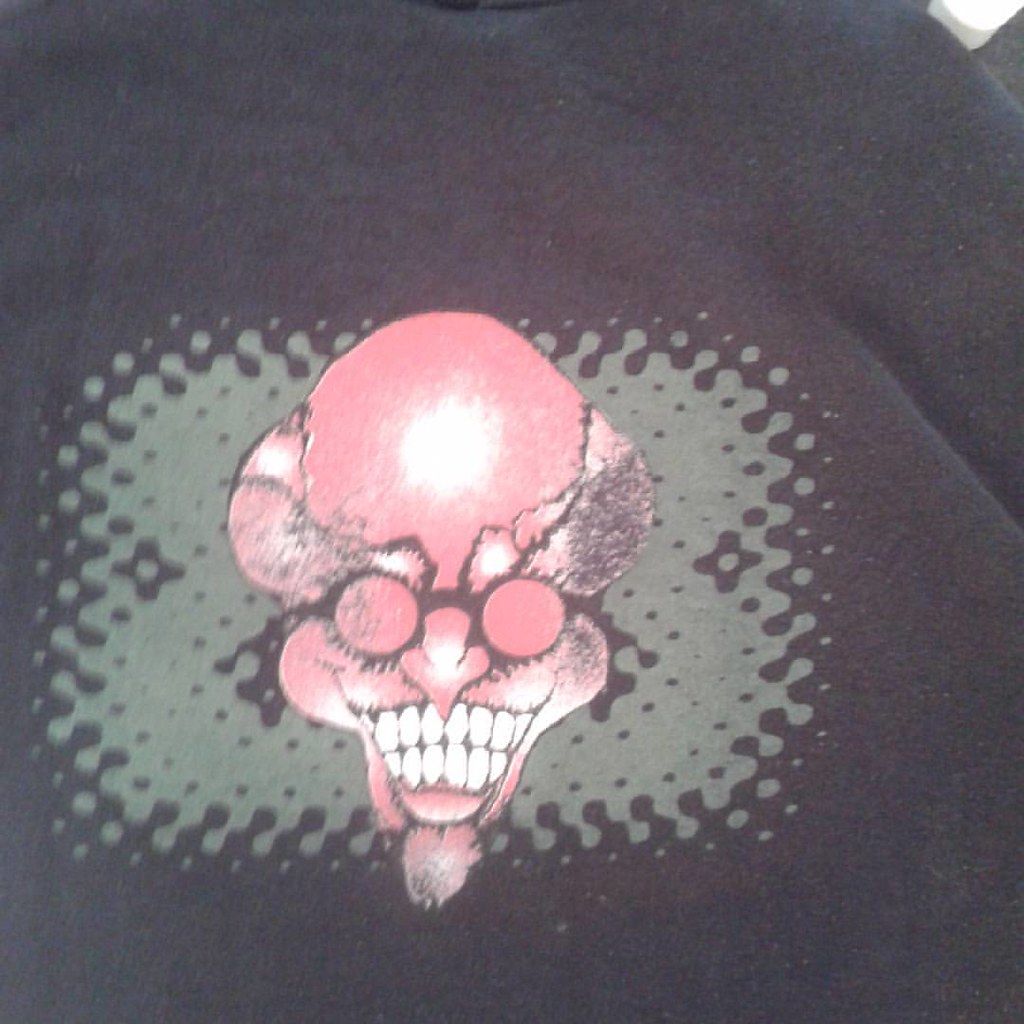This image depicts a graphic printed on a black t-shirt, showcasing the exaggerated portrait of an old man. The man has pinkish, bald skin with a shiny, illuminated spot in the center of his scalp. He wears large, circular black glasses that obscure his eyes, coupled with thick, white eyebrows. His facial features are sharp and exaggerated, including a pointed nose and a very slender, elongated chin. His smile is wide, revealing both rows of large teeth, and a small goatee is visible beneath his bottom lip. His cheeks are prominently round, enhancing the overall caricatured style. Surrounding the man's head is an abstract green rectangular background with black splotchy bubbles, adding a surreal touch to the design.